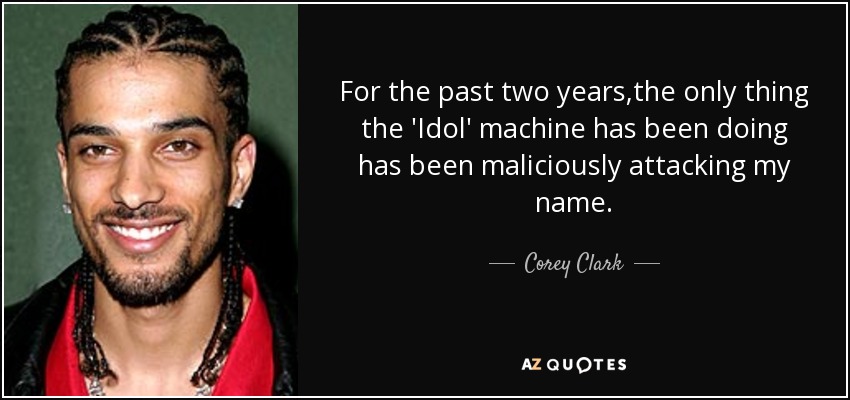The horizontally aligned rectangular image features a picture of Corey Clark on the left side and a solid black background on the right side with centered white text. Corey Clark is a man with slightly dark skin, black eyebrows, a thin black mustache, and a faint beard. He sports a few small stud earrings in each ear and has his hair braided back with thin braids cascading around his neck to the front. He is wearing a red-collared shirt under a black jacket and is smiling broadly, showing his teeth. 

The text on the right reads: "For the past two years, the only thing the idle machine has been doing has been maliciously attacking my name." Directly underneath this quote, there are small dashes on each side of his name, "- Corey Clark -". At the very bottom, the text "AZ QUOTES" is displayed in all caps, with the letter "Z" in orange and all other letters in white.